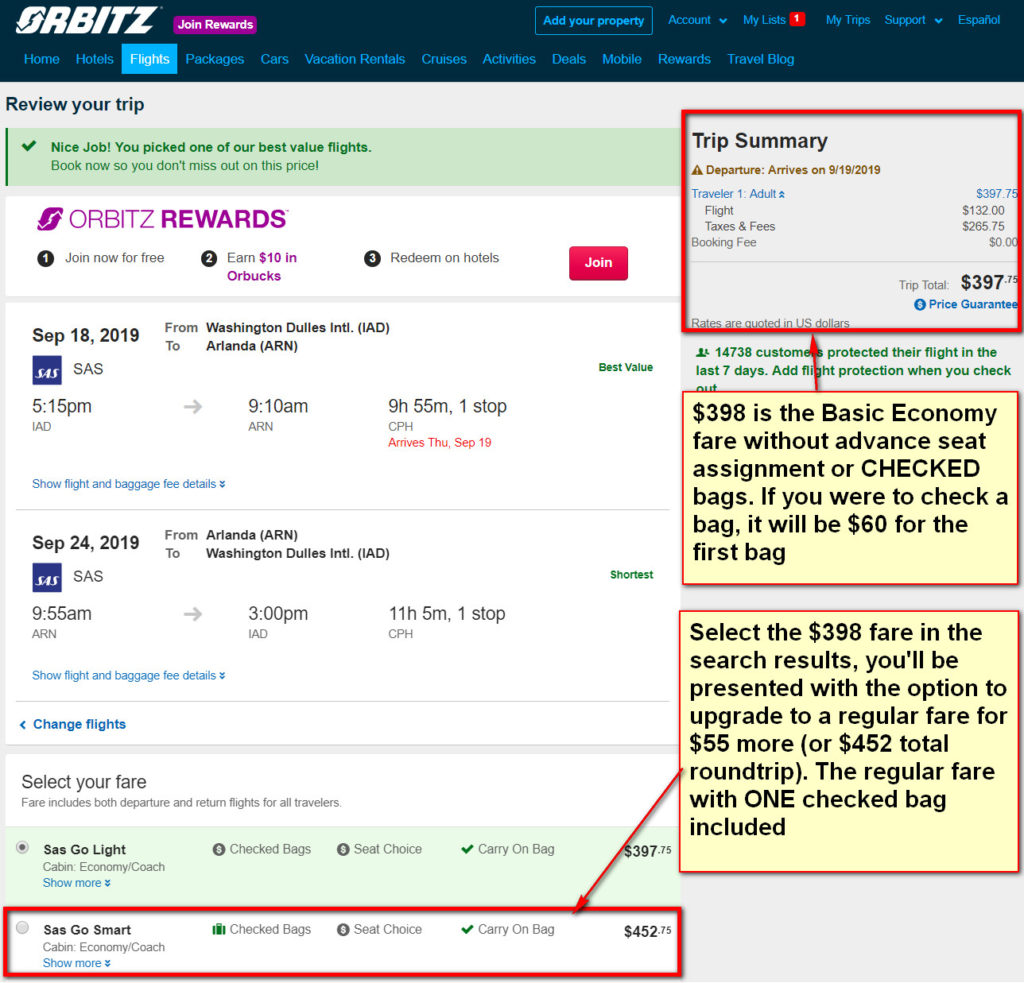This image from Orbitz displays a booking summary for a flight priced at $398 under the basic economy fare, which does not include an advanced seat assignment or checked bags. If you need to check a bag, it will cost an additional $60 for the first one. You are given the choice to select the $398 fare during the booking process. Alternatively, you have the option to upgrade to a regular fare for $55 more, totaling $452 for a round trip with one checked bag included. The trip summary includes:

- Departure and arrival date: September 19, 2019
- Traveler: One adult
- Flight details
- Taxes, fees, and booking fee
- Total trip cost: $397.75

There is also a price guarantee option. The rates are quoted in U.S. dollars. Additionally, it notes that 3A customers protected their flights within the last 7 days, highlighting a total amount of $1,470.